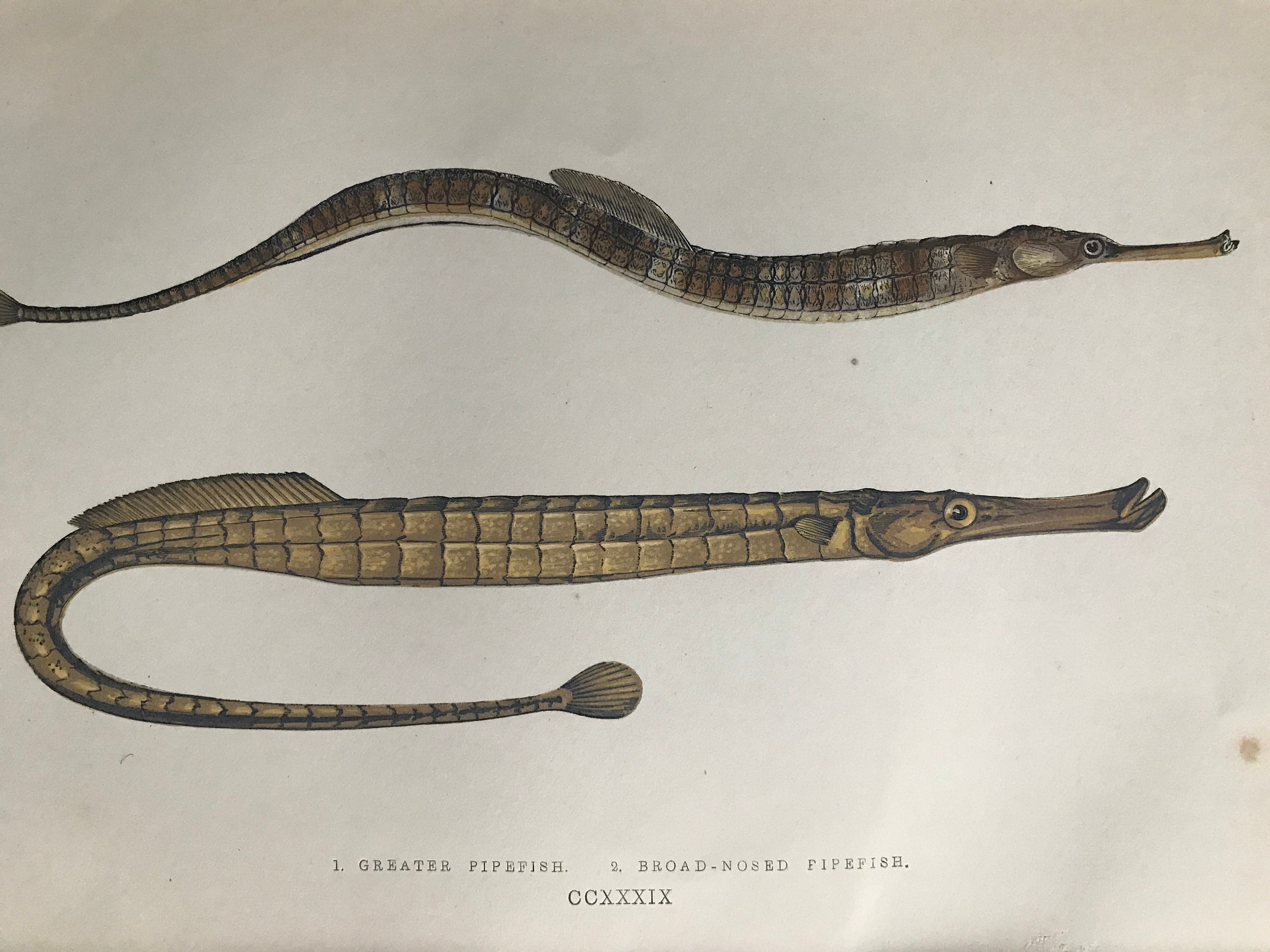The image is a detailed illustration from an aged book page, depicting two fish: the greater pipefish and the broadnose pipefish. These exotic creatures have elongated, slender bodies with distinctive long snouts that evoke a blend between seahorses and eels. Their skin displays earthy tones of browns, grays, and whites, reminiscent of snake skin, accentuated by scales that give them an almost alligator-like appearance. Each fish has a prominent fin on its back, rising from the middle of its body, and tapering down to a flat tail fin. The illustration is accompanied by text specifying “one greater pipe fish” and “two broad-nosed pipe fish,” along with the Roman numerals CCXXXIX (239). The page itself looks quite antiquated, adding to the prehistoric aura of the fish.